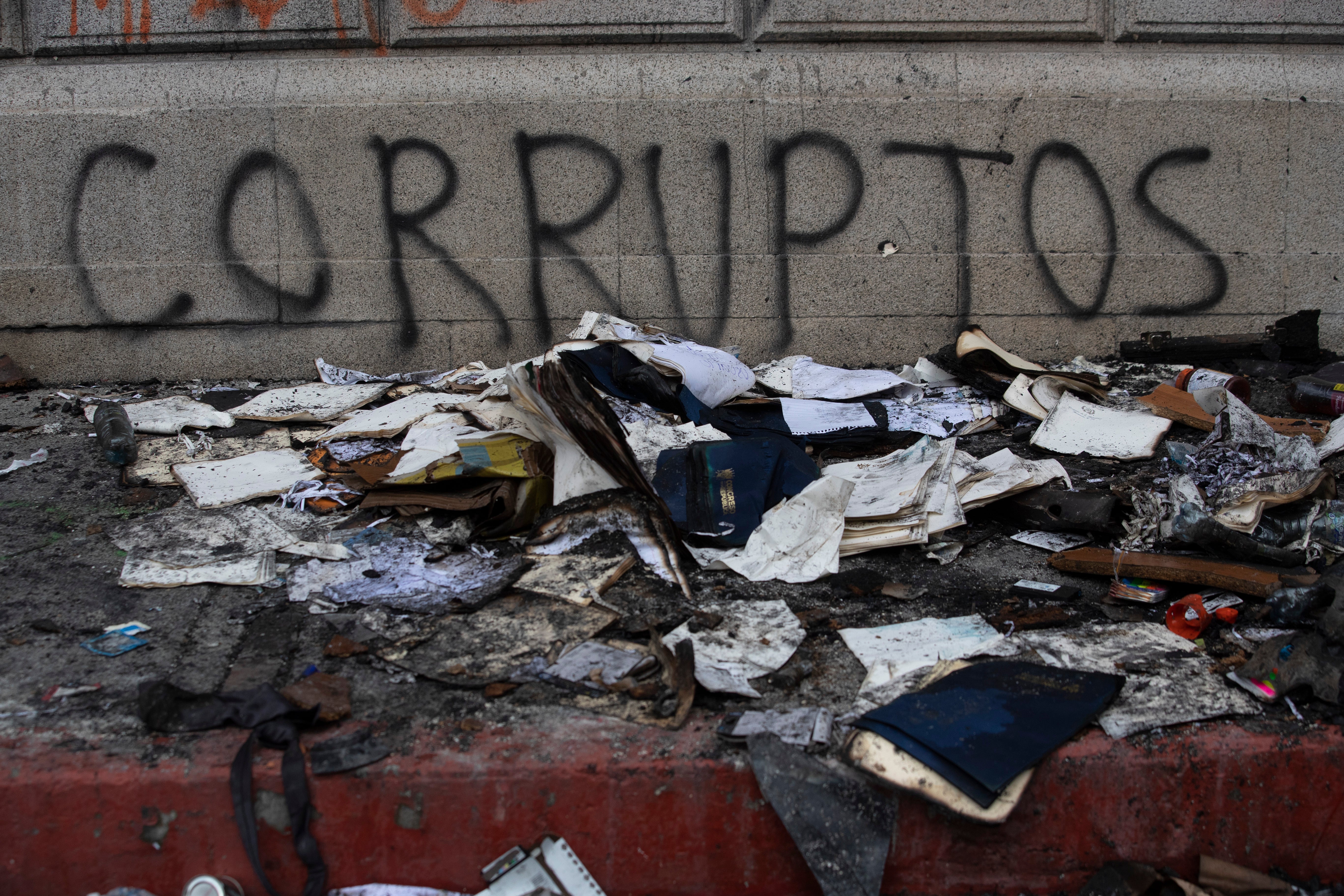Captured under a likely cloudy sky during the day, this outdoor color photograph depicts a grimy urban scene at street level. Dominating the background, a brick or cement wall bears fresh, bold graffiti spelling "CORRUPTOS" in jagged, capital letters. The graffiti stands starkly against the muted and dirty gray tones of the surroundings. In the foreground, at the edge of a sidewalk painted red, lies a large, unsightly pile of trash. Amidst the detritus are scattered documents, binders, napkins, paper pieces, and various other refuse, some scorched and burned, with remnants of bright red, blue, white, and brown contributing streaks of color. This heap of garbage is partially resting against a deep red steel structure that adds to the grimy, dilapidated atmosphere of the scene. The overall impression is one of urban neglect and decay.